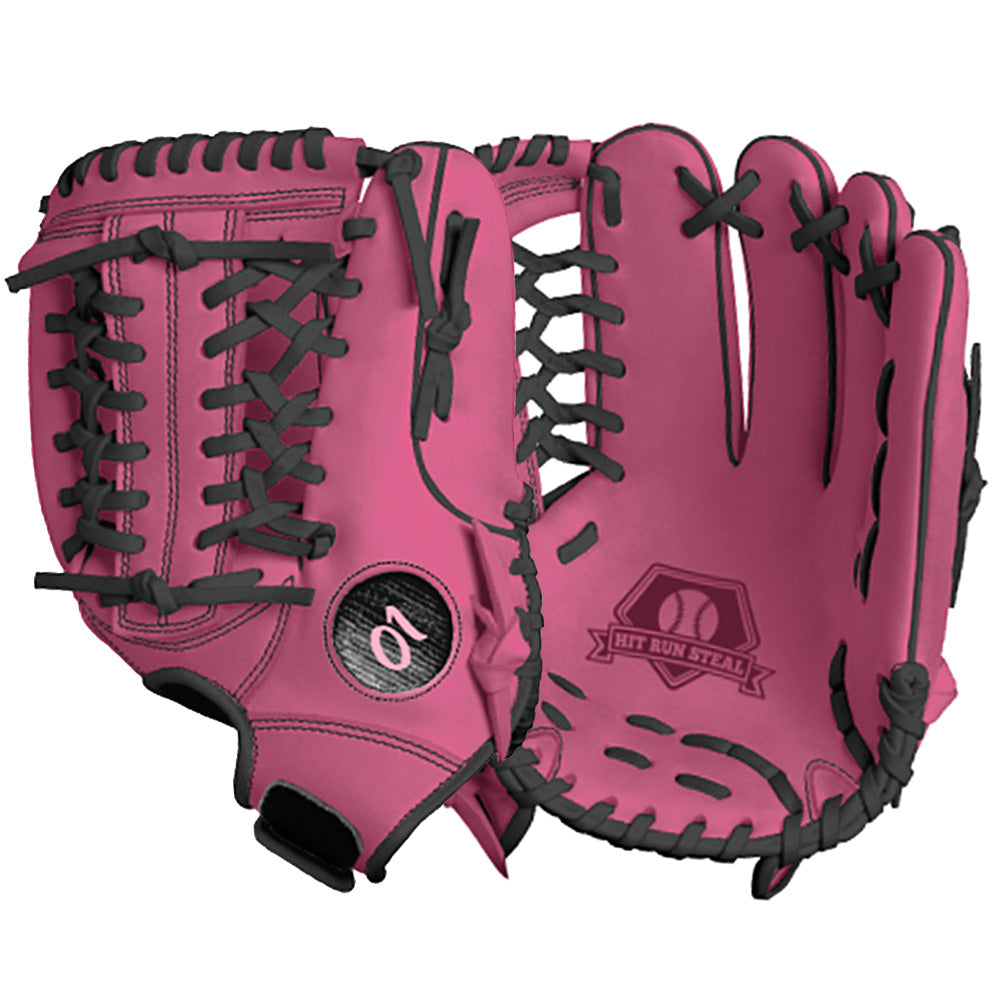The image showcases a product set against a plain white background, prominently featuring a pair of pink baseball gloves with intricate black lacing. The gloves are positioned centrally, slightly overlapping, showcasing different angles. On the left glove, the outer side is visible, displaying a black circle near the bottom with the number "10" inscribed. The lacing forms an elaborate woven pattern. The right glove is shown with the palm facing outward, highlighting an illustration in the center featuring a pentagonal logo with a baseball figure inside. Beneath this logo is a banner with the inscription, "Hit Run Steal." Both gloves are made of pink leather and are detailed with black ties, emphasizing their stylish and functional design as baseball equipment.